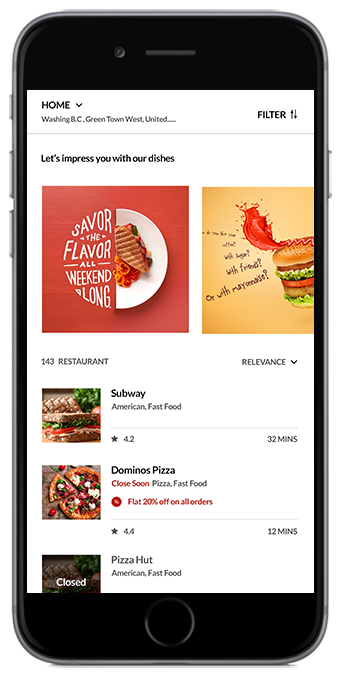The phone screen displays a predominantly black background. Centrally, there's a white rectangle featuring multiple text elements. At the top in bold black print, it reads "Home." Just below, in the same black print, appears "Washington, D.C., Greentown, West, United." Adjacent to this is a filter option. Further down, in a striking red rectangular background with white text, it states, "Let's impress you with our dishes." Halfway through the red rectangle, more white print enthusiastically reads, "Savor the flavor all weekend long." 

Next to this, there is an image of a plate of food against a black square background, cutting off part of the red rectangle. Beside the plate, within a partially obscured box, there’s tiny print that is mostly illegible. The visible part transitions into larger print, posing a question that might say, “with fries?” or “with mayonnaise?” accompanied by a picture of a burger.

The layout returns to white space, where it shows "143 Restaurant" followed by the text “relevance.” At the bottom, the screen presents the option to choose popular food chains: Subway, Domino's, or Pizza Hut.